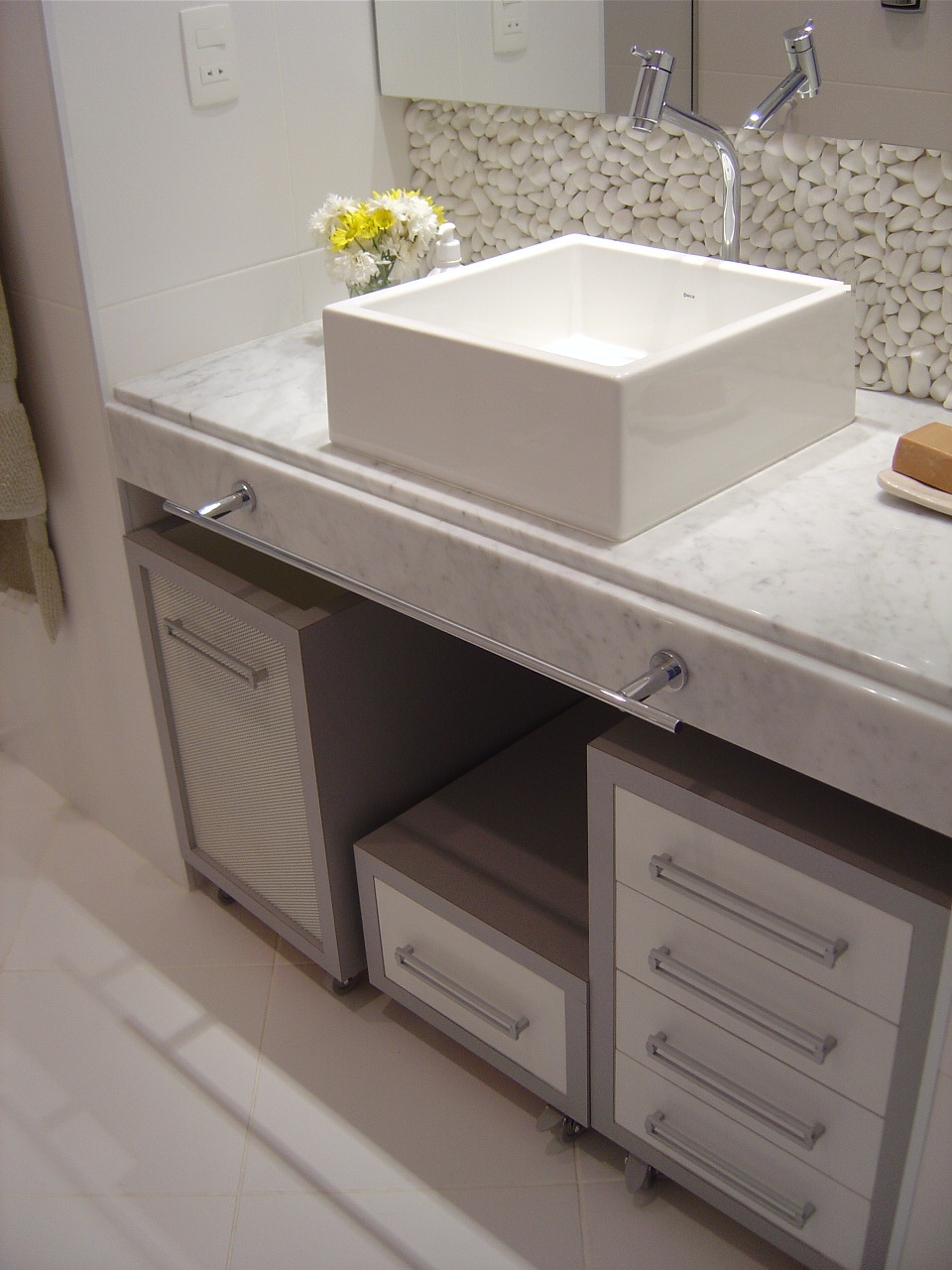The image displays a meticulously organized bathroom predominantly adorned in shades of gray and white, save for a splash of color provided by a small bouquet of yellow and white flowers positioned in the top right corner. A light switch is situated adjacent to the flowers, near the upper area of the image, and it is also reflected in a sliver of a mirror nearby. Central to the scene is an elegant, raised white porcelain sink with a sleek square design, topped with a silver faucet.

Next to the sink rests a soap dish holding a brown bar of soap, neatly placed on the marble-colored counter. Beneath the counter, a drawer with a marble finish and a silver pull handle stands prominently. Below this main drawer, multiple pull-out drawers, also featuring a gray and silver color scheme, are visible, with their tops showcasing a distinct brown hue. The floor comprises pristine white tiles, and in the upper corner, a hint of a robe hangs, subtly suggesting the room’s purpose and the potential for relaxation it offers.